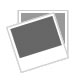The image features a package of moth balls positioned on a chipping white countertop on the left side. The prominently blue and white package, accented with red and black text, clearly states "moth balls" and details its efficacy: "kills clothes moths, eggs, and larvae." It specifies usage for airtight containers and storage closets, treating up to 50 cubic feet. The package contains two white packets filled with small, gray balls, and is adorned with a small American flag, indicating it’s made in the USA with U.S. and imported materials. The protective wrap caution advises no direct skin contact. Partial text at the bottom hints at "convenient" and "active ingredient," although it's cut off. Next to the package, a blurry box bears additional usage instructions that are not legible.